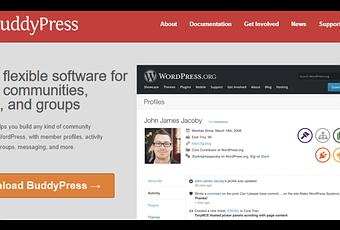The image depicts a cropped screenshot of a web page. The top navigation bar is partially visible, showing the text "uddPRESS" with menu options for "About," "Documentaries," "Get Involved," "News," and "Support" — though the "T" in "Support" is cut off due to the cropped nature of the image. 

Below the navigation bar, the main header reads "Flexible software for communities, groups," suggesting a web page dedicated to promoting software designed for building and managing online communities. Beneath this header, there is additional text that is partially obscured but mentions features like "member profiles," "activity," "maps," "messaging," and more. 

An orange button labeled "Upload BuddyPress" with an arrow icon is prominently displayed, likely encouraging users to download or install the software.

To the right of this section, there is a profile snippet from WordPress.org featuring a man named John James Jacoby. His profile includes a photo of a white man with brown hair and glasses, accompanied by text and several icons, the details of which are not discernible due to the image quality.

Overall, the image appears to be a cropped screenshot from a web page related to BuddyPress, a WordPress plugin aimed at creating and managing online communities.